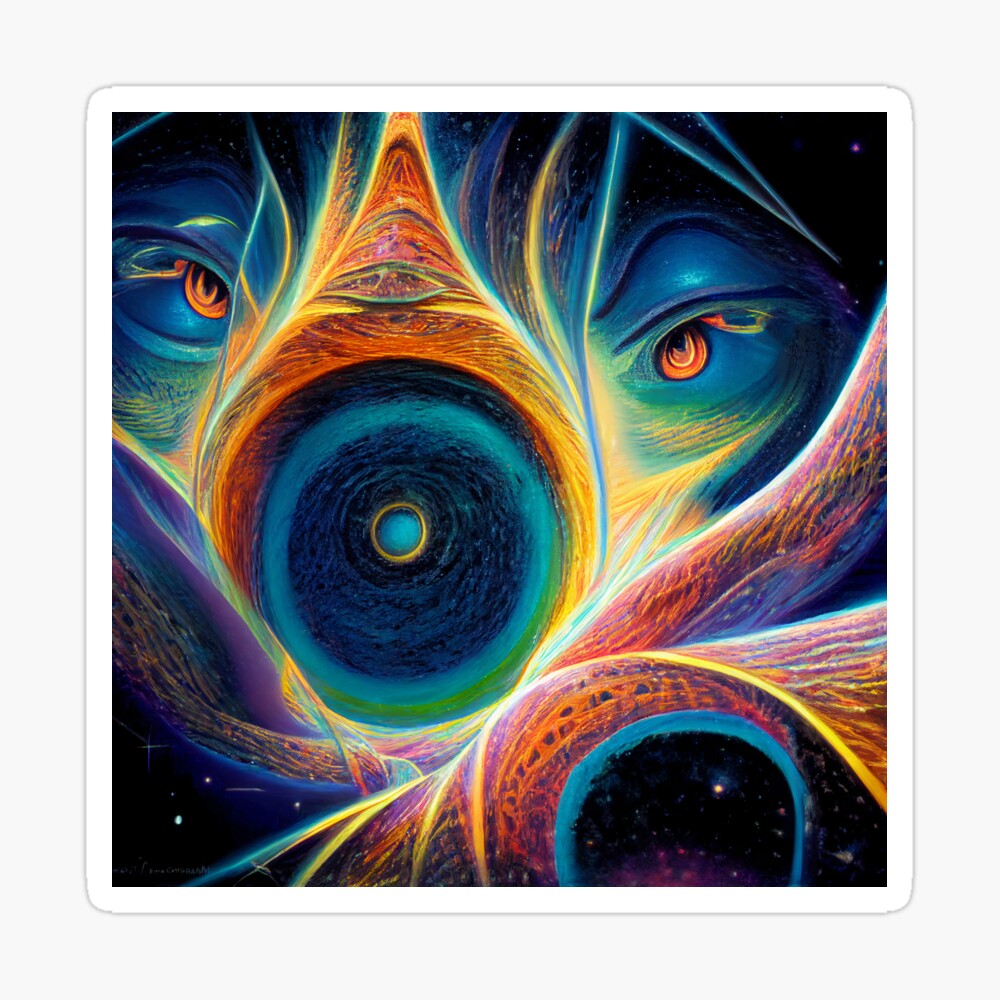This intricate and vibrant piece of abstract artwork, framed in white, appears to be a computer-designed graphic filled with swirling shapes and rich colors. Dominated by shades of blue—from deep to royal—the design is reminiscent of the peacock's tail. On closer inspection, the intricate patterns reveal a scene with two heavily lidded, blue-orange eyes flanking either side of a rounded, red and blue snout, evocative of an animal peering through foliage. The eyes, set against a backdrop of swirling oranges, yellows, tans, greens, and strokes of purple, suggest a mysterious creature in a cosmic setting. At the center of the composition is a large circle filled with gradient shades of blue, giving it depth and focus. This circle, embraced by a cornucopia-like structure made of warm hues, adds to the dynamic, flowing tapestry-like feel of the artwork. The dark background, sprinkled with star-like points, enhances the impression of a scene unfolding in the expanse of space, making the whole piece a fascinating blend of organic and celestial aesthetics.